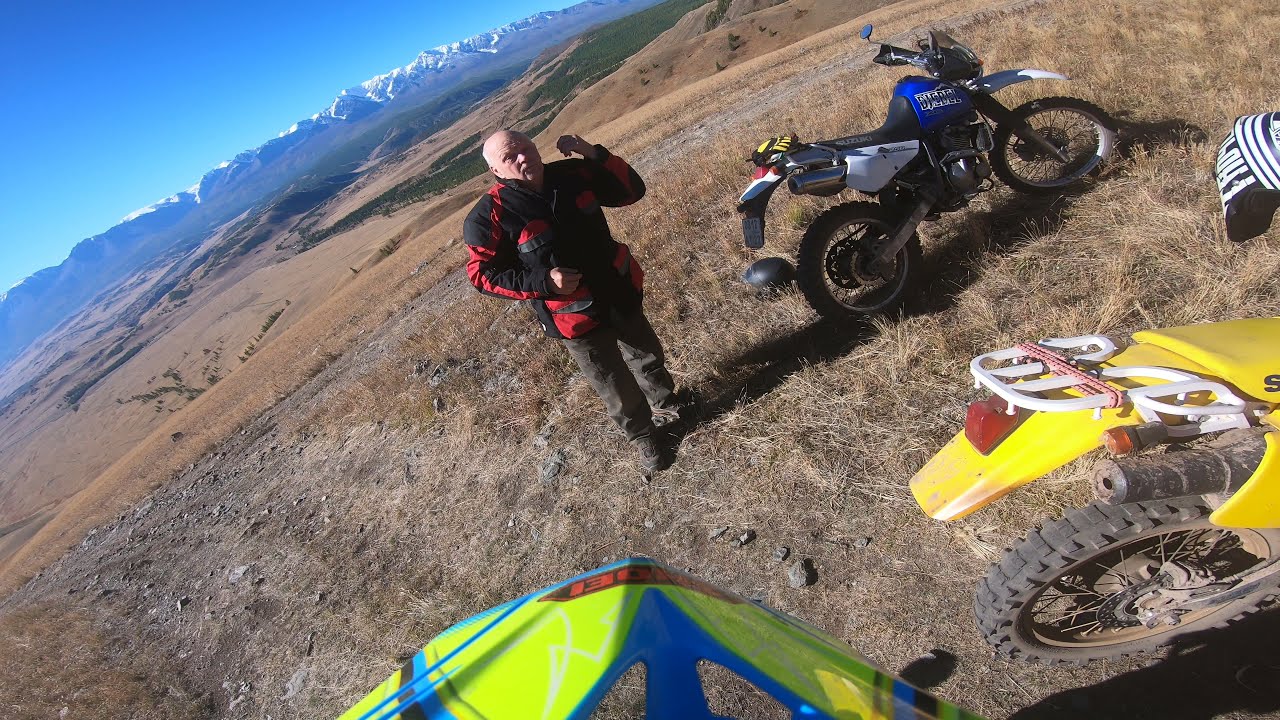In the image, an older, balding man with gray hair stands in a scruffy, beige desert landscape, which features rocky, colorless terrain. He is wearing a red and black jacket, buttoned up, and dark gray slacks. Standing beside him, to his right, is a blue motorcycle, which appears to have a black and white body. Partially visible in the foreground is another motorcycle, yellow with a white rail on the back, revealing a tire and parts of an additional vehicle. In front of the man, there is a plastic tent-like structure with a mixture of yellow and blue colors on it. The background shows a vast expanse of desert leading to distant hills, and further still, snow-capped mountains under a blue sky filled with puffy white clouds. The entire photograph is taken at a slight angle, giving a unique perspective to the scene.